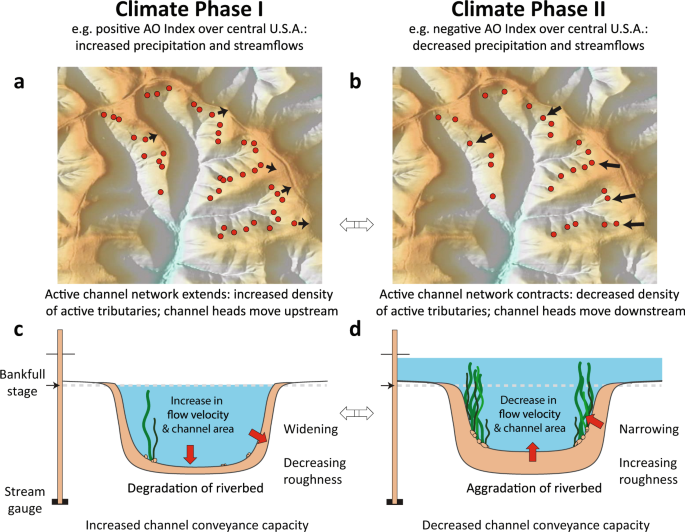The image consists of four distinct panels labeled A, B, C, and D, each with a pictograph and accompanying text, focusing on climate phases and their impact on streamflows and riverbeds. Panel A, labeled "Climate Phase 1," features a topographical map of the central USA with white, yellow, and gray shades plus red spots, and the text "Positive AO Index over Central USA: Increased Precipitation and Streamflows, Active Channel Network Extends, Increased Density of Active Tributaries, Channel Heads Move Upstream." Panel B, labeled "Climate Phase 2," presents a similar topographical map but highlights a "Negative AO Index over Central USA: Decreased Precipitation and Streamflows, Active Channel Network Retracts, Decreased Density of Active Tributaries, Channel Heads Move Downstream." Panel C, showing a diagram of a water-filled channel, reads, "Bankfull Stage Stream Gauge: Increase in Flow Velocity in Channel Area, Degradation of Riverbed, Increased Channel Conveyance Capacity." Panel D features a similar pictograph to Panel C and is captioned "Aggredation of Riverbed, Decreased Channel Conveyance Capacity." Overall, the image illustrates the changes in river and stream behaviors under different climate conditions, emphasizing the alterations in water flow and riverbed conditions.